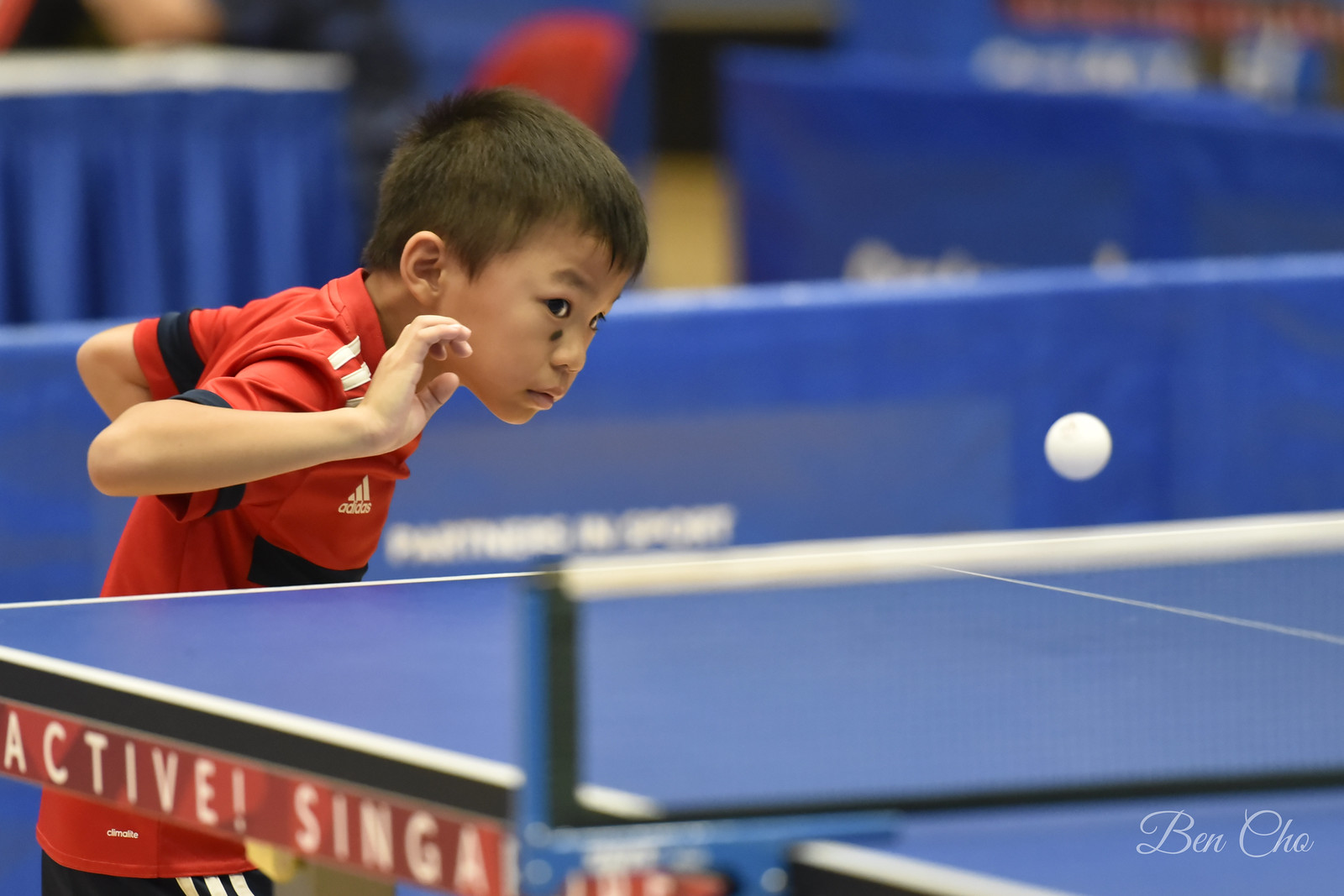In a vivid landscape-oriented photograph, a young Asian boy, possibly five years old, is deeply engrossed in playing ping-pong. He is dressed in a red, black, and white Adidas shirt with matching black shorts. The boy stands at the center-left of the image, poised at a blue ping-pong table with the white ball captured mid-air to the center-right. His right hand is raised, eyes intensely following the ball, while his left hand, somewhat obscured from view, presumably holds the ping-pong paddle. A distinctive mole or birthmark is visible under his right eye. An inscription along the table's side reads "Active Singapore," hinting at the location, and in the bottom right corner, the script "Ben Cho" suggests the photographer's name. The background features additional blue-draped ping-pong tables and a red chair, adding context to the scene.